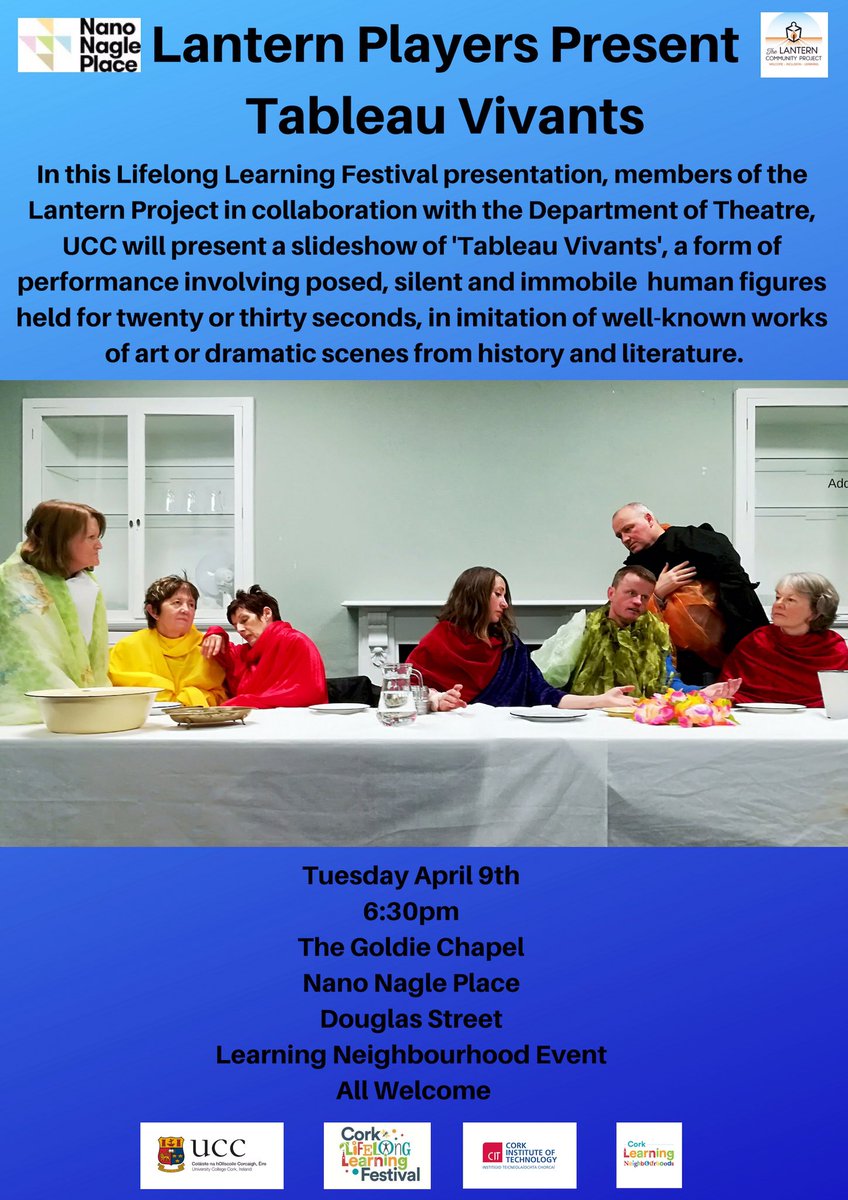The image is an advertisement for an event presented by the Lantern Players called "Tableau Vivants." At the top, a blue rectangular banner features the black text: "Lantern Players Present Tableau Vivants." The text explains that during this lifelong learning festival presentation, members of the Lantern Project, in collaboration with the Department of Theater, University College Cork (UCC), will showcase a slideshow of Tableau Vivants. This art form involves posed, silent, and immobile human figures held for 20 to 30 seconds, mimicking famous works of art or dramatic historical and literary scenes. The photograph below this description depicts people at a long table covered with a white tablecloth, arranged to recreate Leonardo da Vinci's iconic painting, "The Last Supper." The scene is set against a light green-gray wall, featuring built-in glass shelves with white frames and a white fireplace mantle in the background. At the bottom of the image, another blue rectangular section of black text details the event specifics: "Tuesday, April 9th, 6.30 p.m., The Goldie Chapel, Nano Nagel Place, Douglas Street, Learning Neighborhood Event, All Welcome." Accompanying this information are the logos of the event sponsors: University College Cork (UCC), Cork Lifelong Learning Festival, Cork Institute of Technology, and Cork Learning Neighborhoods. This event appears to be part of the Cork Lifelong Learning Festival and is open to everyone, suggesting a welcoming and inclusive community gathering in Ireland.